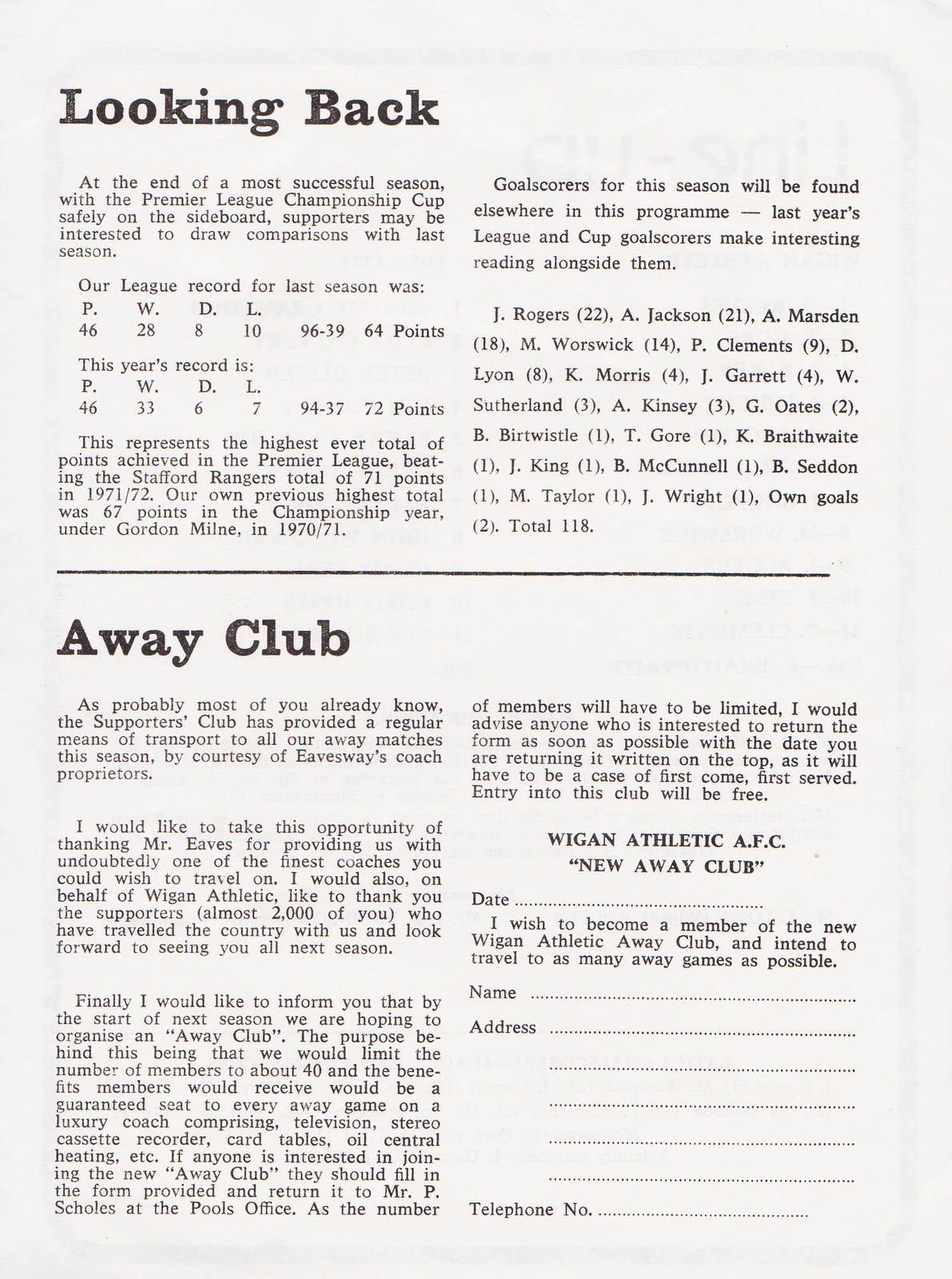The image displays a newspaper or magazine clipping featuring black text on a white background, possibly in Arial or Times New Roman font. The paper is thin, allowing a glimpse of the reverse side. The page is divided by a horizontal break line. The upper section reflects on a successful Premier League season, noting the team’s record-breaking points total, which surpassed the previous highest of 71 points set by the Stamford Rangers in the 1971-72 season. It includes detailed comparisons with the past seasons and mentions the goal scorers, whose names appear elsewhere in the publication. At the bottom, there is a section titled 'Away Club' presented in two columns, where the team extends gratitude to their around 2,000 supporters and highlights the importance of their assistance. It also provides a form for readers to join the New Wegan Athletic Away Club, offering opportunities for travel to away games, asking for contact details including name, address, and phone number.